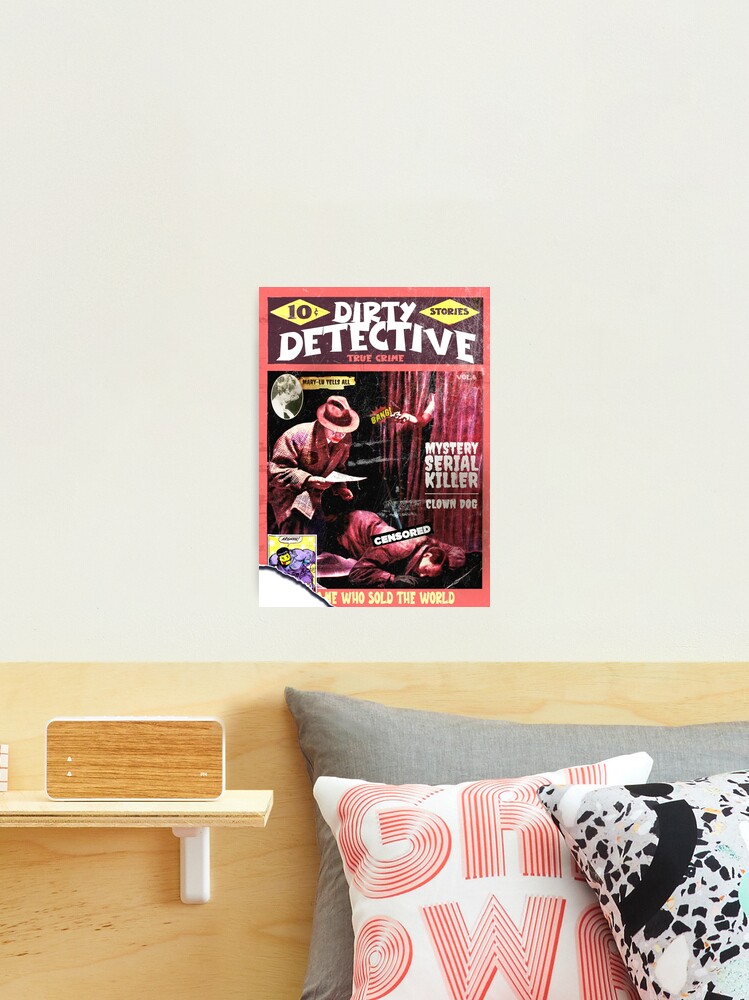The image depicts a vintage magazine cover titled "Dirty Detective," priced at ten cents, with text presented in white capital letters. The words "Ten Cents" and "Stories" are featured within yellow diamonds flanking the title. Beneath the title, it reads "Dirty Detective True Crime." The cover showcases a 1940s-style detective in a trench coat and fedora, leaning over a dead body and reading a piece of paper, with the word "Censored" emblazoned across the body. Additional text on the cover includes "Mystery Serial Killer" and "Clown Dog." In the background, there is a hand reaching through a curtain, holding something out to the detective. The setting seems to be a bedroom, with the magazine cover attached to a beige wall above three pillows—one dark gray, one red with partial text reading "GRI something W something," and a black and white pillow. To the left of the pillows is a wooden shelf with what appears to be a wooden clock.